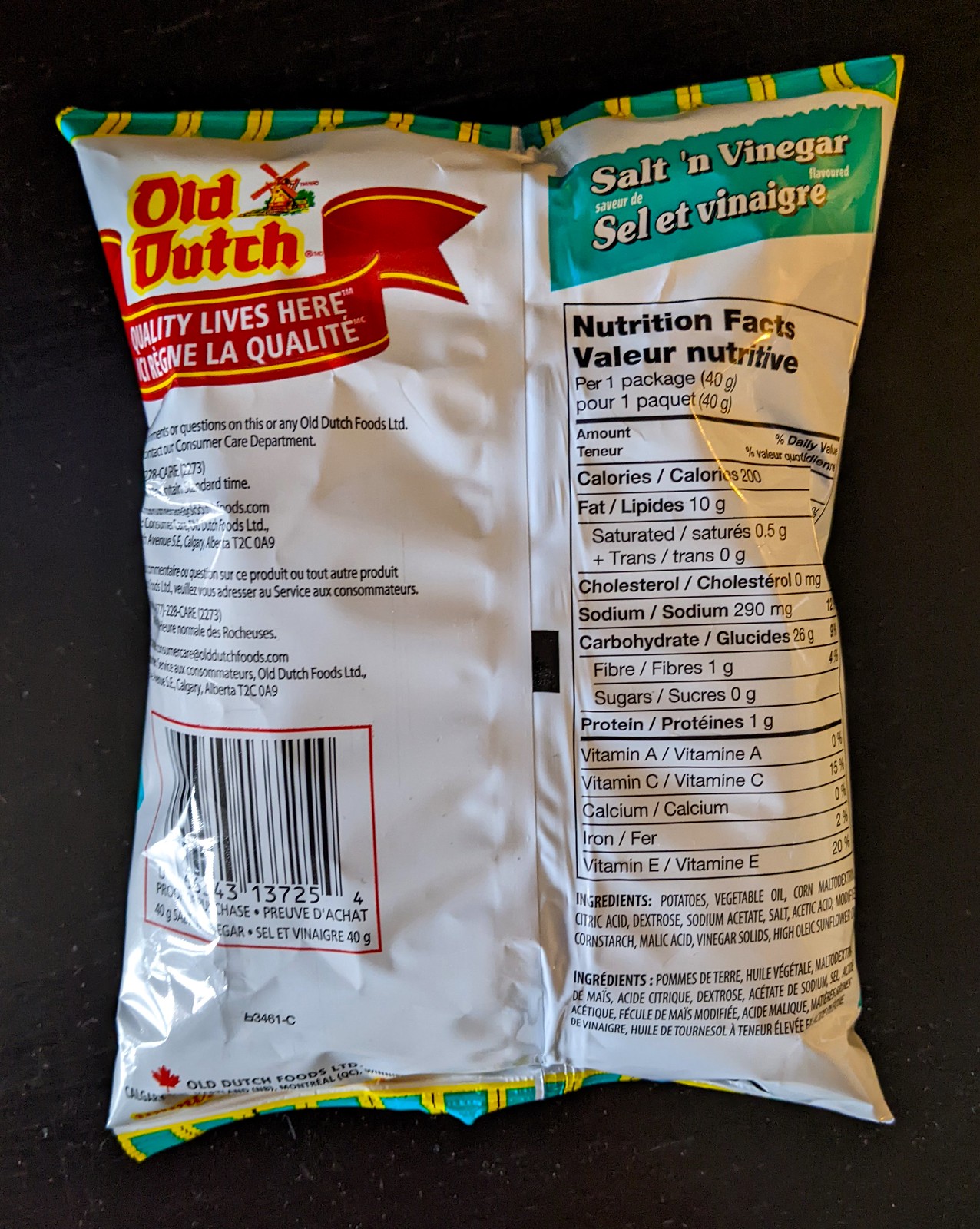This image features the back side of a bag of Old Dutch brand Salt and Vinegar flavored chips. The top left-hand corner of the bag showcases the Old Dutch logo along with the slogan "Quality Lives Here." Dominating the right-hand side is a long, rectangular table presenting the nutrition facts, detailing the amount of calories, fat, cholesterol, sodium, carbohydrates, sugars, protein, vitamins, calcium, and iron per serving. Directly below this table, the ingredients are listed. The barcode, white and black with a red rectangular outline, is located in the bottom left-hand corner of the bag. The primary color of the bag is white, with teal and yellow accents along the edges, adding a pop of color to the overall design.